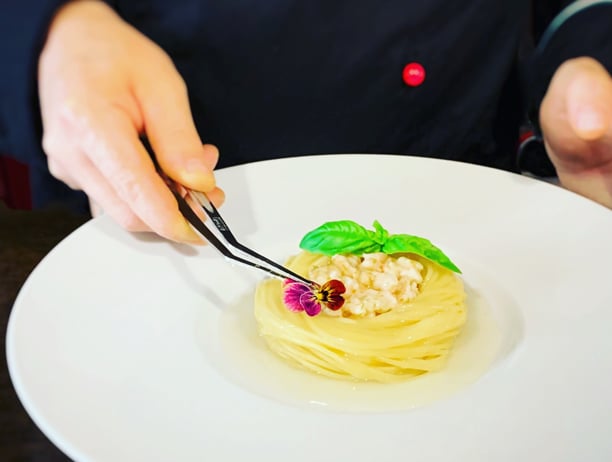In this detailed color photograph, we see a chef meticulously plating a high-end dish in a landscape orientation. The subject is a sophisticated creation centered on a white, round platter with a slight indent meant to keep food contained. This gourmet presentation features a nest-like arrangement of creamy-colored chow mein noodles, intricately wound together. At the center of this nest lies a hollowed-out area filled with a creamy white substance, resembling the core of a piece of fruit. Adorning this culinary art are delicate garnishes: two vibrant green leaves on the top right and a tiny purple flower blossom, which the chef is delicately placing with a pair of silver mini tongs. The background reveals part of the chef, cropped off at mid-chest, dressed in a black shirt with a distinctive red button. The colors throughout the image are vivid, with the stark contrast of the white plate, the yellow noodles, the green leaves, and the purple flower, all coming together to create an eye-catching and appetizing visual experience.